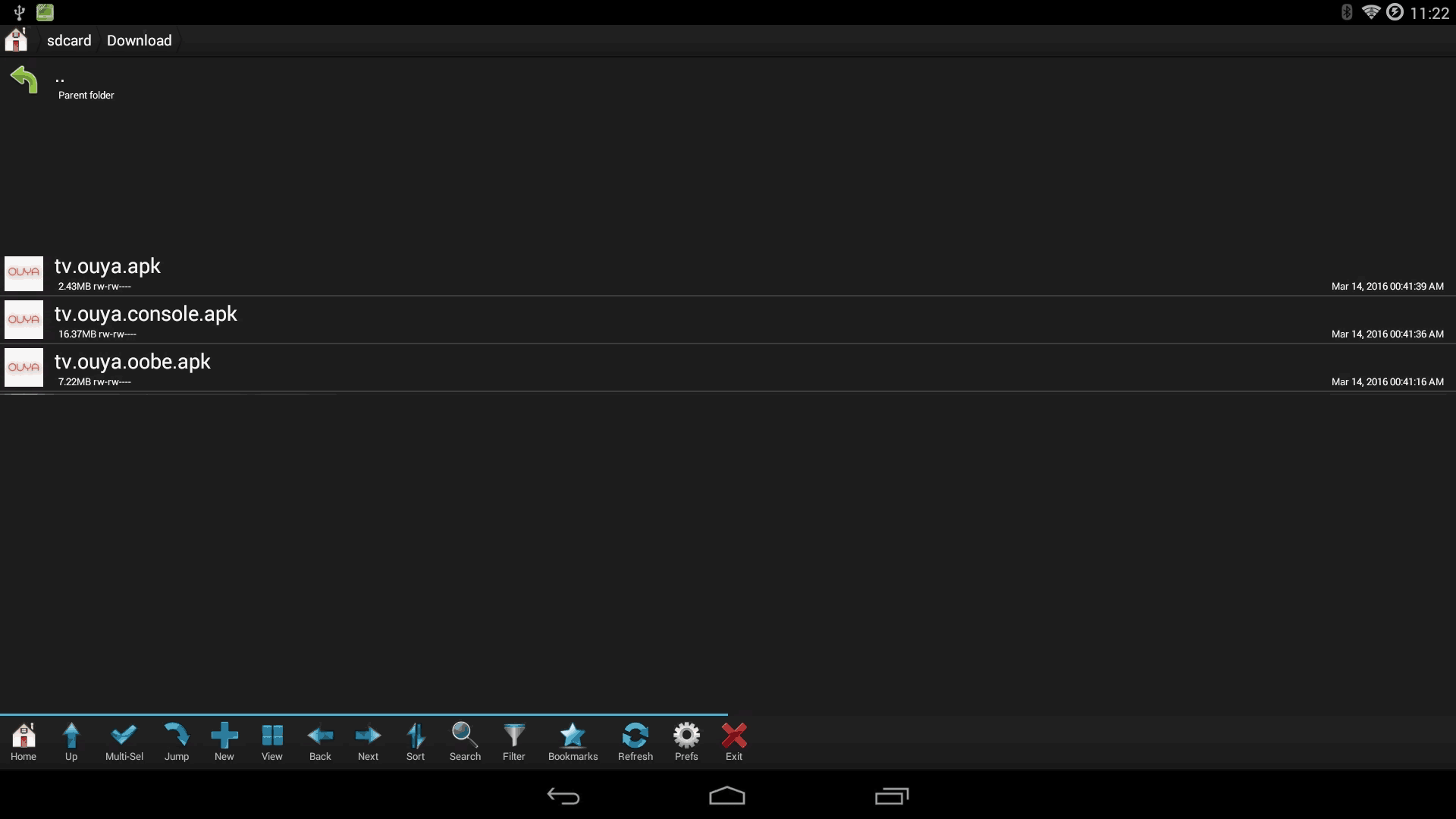This screenshot appears to be from a tablet in landscape orientation. The bottom center of the screen has a home icon, indicative of a tablet interface, flanked by a back icon on the left and a tabs icon on the right. 

The main display features white and blue text on a black background. At the top right of the screen are a series of small, grayed-out icons: a Bluetooth indicator, a Wi-Fi signal indicator, a lightning bolt within a circle, and the current time displayed as 11:22. To the far left, there is a USB indicator next to a green square. 

Beneath these icons is a row containing a home icon, followed by the words "SD card" and "Download". Further below, a green arrow pointing left is accompanied by the white text "Present Parent Folder."

Central to the image are three rows of applications, each marked with the OUYA logo and a date on the far right, suggesting the download dates for these apps. 

At the bottom, above the navigation icons, a series of function icons are displayed: a white home icon, and then blue icons including an up arrow, a check mark, a right-pointing arrow, a plus sign, a grid, left and right arrows, a lightning bolt, a magnifying glass (or possibly a question mark), a filter option, a star, a blue refresh button, a gray cogwheel, and a red X. 

This detailed layout suggests a comprehensive view of a tablet's interface, highlighting both functional elements and application organization.